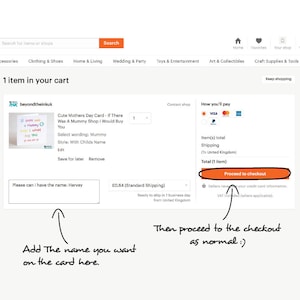The image displays a small, square-shaped interface, likely from a website viewed on either a computer or a smartphone. At the top, there's a search bar for inputting queries, with an orange button labeled "Search" in white letters to its right. Adjacent to this, on the upper right, are several icons including a "Home" button, a heart symbol for favorites, and another actionable icon.

Below these top elements, there are clickable headings in black font, categorized under different interests such as clothing and arts. The main section features a light gray background with the text "One item in your cart" prominently displayed in bold black letters. Below this, there is a detailed view of the cart item, including an image, a title, a brief description, and a quantity adjustment option.

On the right-hand side of the item details, there are payment options, showcasing various credit card icons and relevant information for proceeding with the purchase. A prominent orange button labeled "Proceed to Checkout" is circled in black, which appears to be an annotation made after the screenshot was taken.

At the bottom, handwritten notes instruct the user to "Add the name you want on the card here," accompanied by an arrow pointing to a white input box. Another note reads, "Then proceed to the checkout as normal," followed by a small smiley face and an arrow pointing back to the circled orange button.